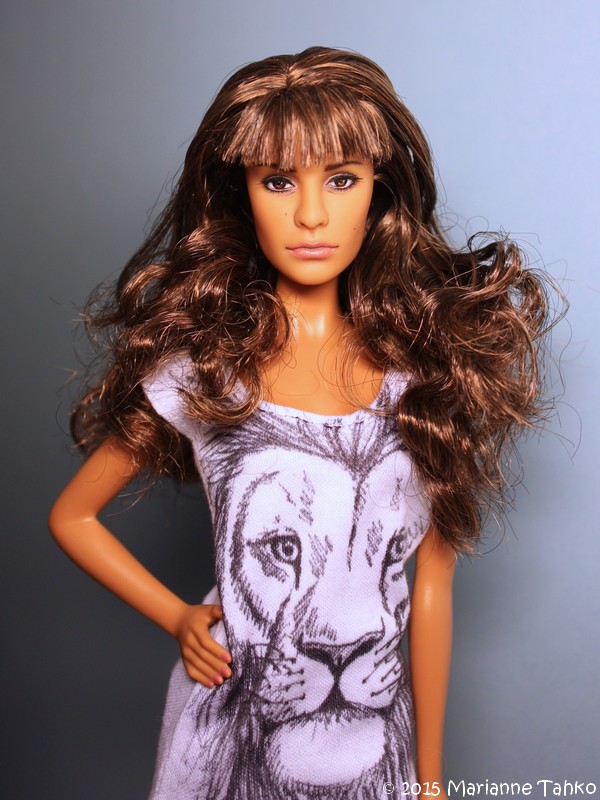The image depicts a doll with a tanned complexion, resembling figures like Penelope Cruz or Catherine Zeta-Jones, with distinct features, including a slightly wider nose and eyes set further apart. The doll has long, dark brown, curly hair with bangs. She is dressed in a white t-shirt dress that prominently features a lion's face design covering almost the entire dress. The lion's face is predominantly black, contrasting with the white dress. The doll adopts a confident pose with her right hand placed on her hip and her other hand resting at her side, gazing directly towards the camera. The background transitions in shades of gray, darker at the bottom left corner and getting lighter towards the top right, giving it an ombre effect. Additionally, the bottom left corner of the image contains the text "2015 Marianne Tackle," signifying the copyright details. The setting is well-lit, enhancing the clarity and color of the overall image.